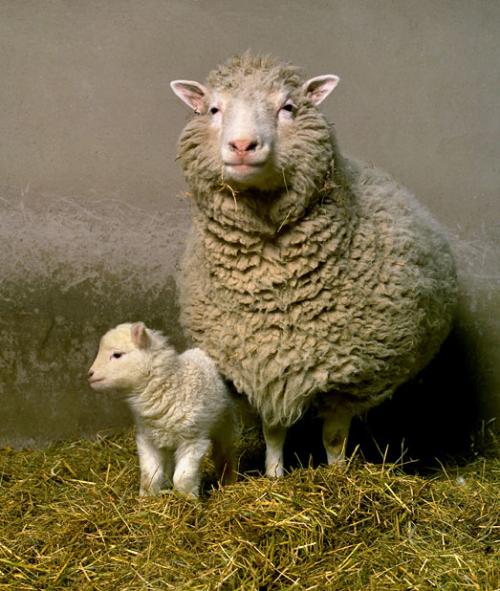The color photograph captures a poignant moment between a mother sheep and her lamb inside a rustic building with a concrete wall in the background. The floor beneath them is strewn with a mix of brownish-green hay and grass. The mother sheep is notably large, with a dingy, wool-covered body that hints at grayish to beige tones, punctuated by a bright pink nose and strikingly white ears. Positioned below and to the left is the lamb, a stark contrast in its pure white coat, with a black nose. The mother sheep gazes directly into the camera while the lamb looks off to the left. This simple yet eye-catching image highlights the textural richness of the sheep’s wool against the muted gray and brown environment, creating a serene and captivating scene.